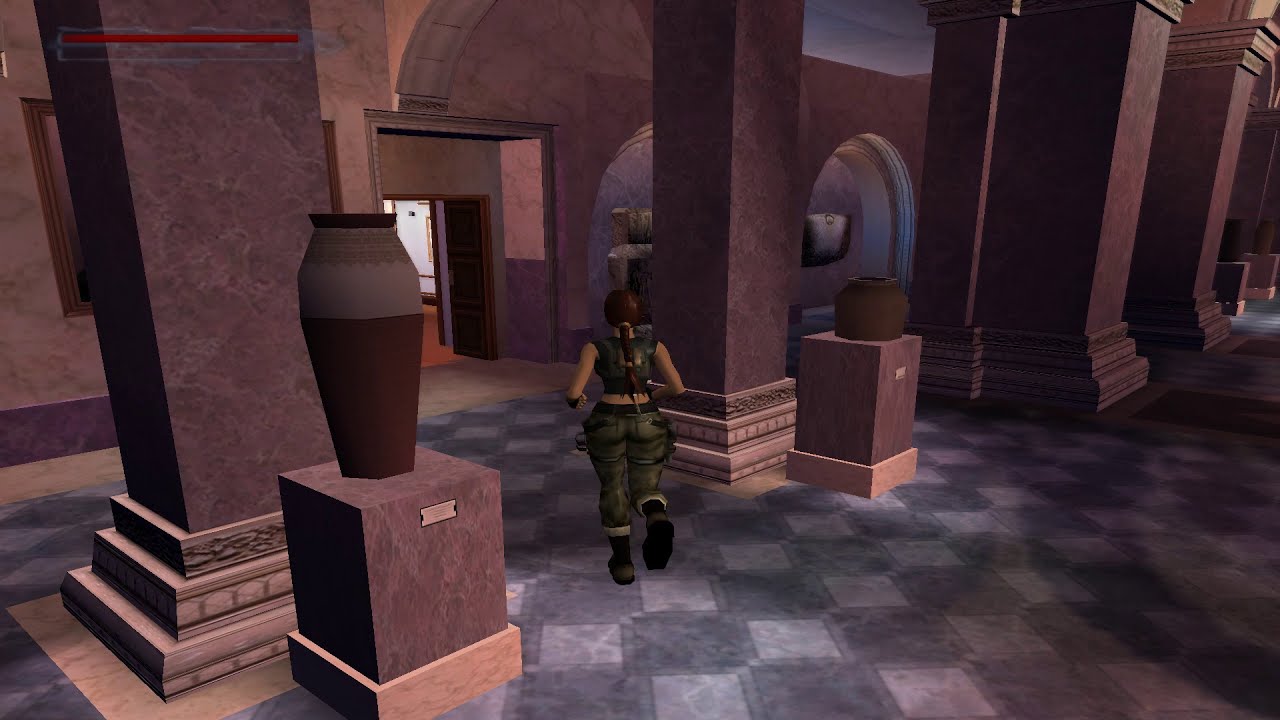This is a screen grab from an old-school video game, likely one of the classic Tomb Raider titles, showcasing the pixelated, blocky graphics typical of the era. The image features the back profile of a woman, probably Lara Croft, distinguished by her brown ponytail, camouflage crop top, camouflage pants, and combat boots. She is captured mid-motion, running through what seems to be a grand palace or museum. The floor beneath her is patterned with black and white marble tiles, and the space is lined with square, rectangular columns. On top of large brown cubes flanking these columns are concrete vases. In the upper left-hand corner of the image, there is a player interface with two bars; one is a red health meter that decreases as the character takes damage, while the purpose of the other remains unclear. The overall visual quality of the image is somewhat pixelated, evoking a nostalgic feel reminiscent of older video game graphics.